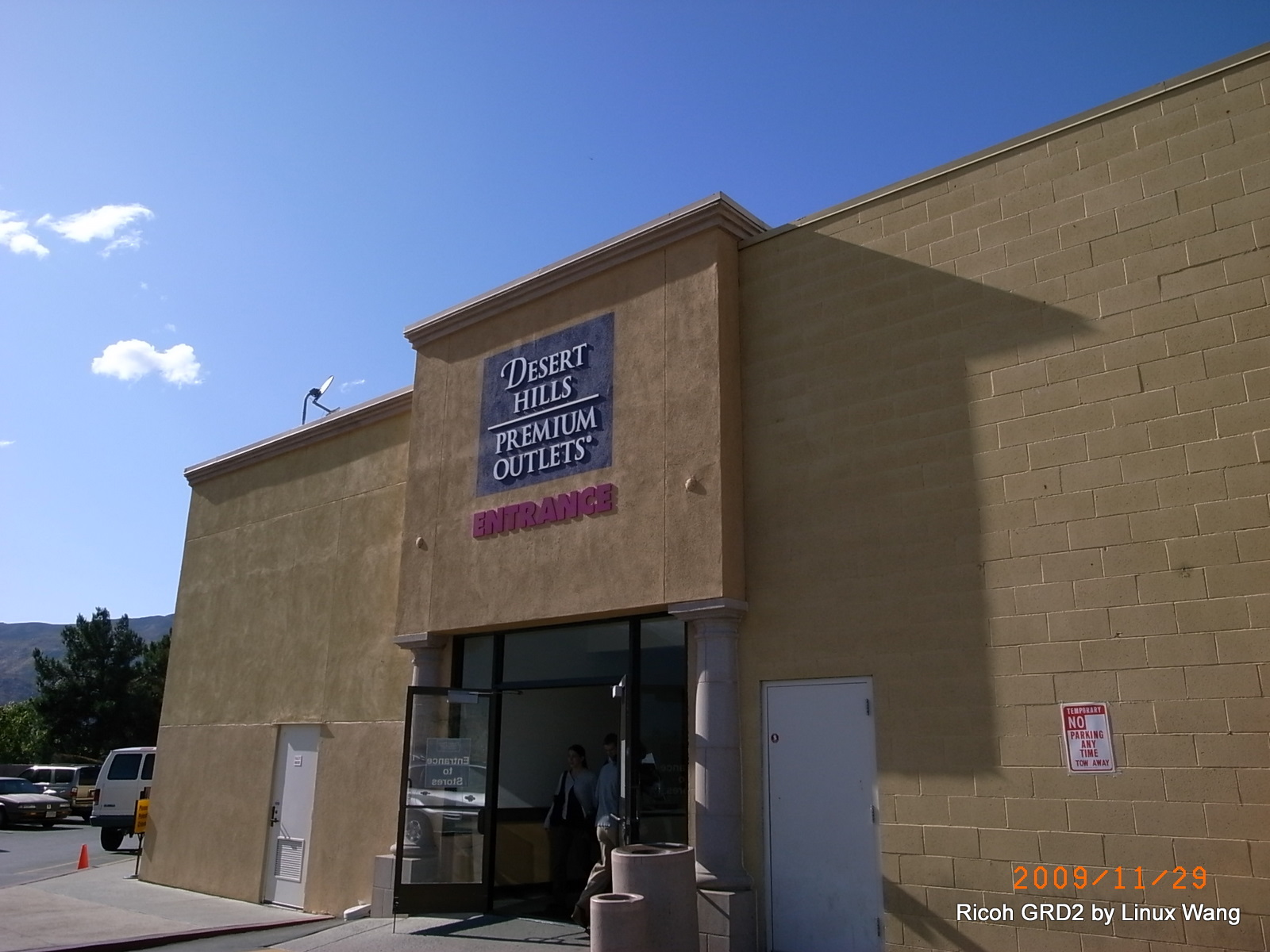The image features a close-up of a brick building, painted brown, showcasing the doorway and the adjacent left side of the building. Prominently displayed at the top of the doorway is a black square sign with white lettering that reads "Desert Hills Premium Outlets," while directly below it, the word "Entrance" is inscribed in red. The entrance itself consists of two glass doors that are open, set within a sturdy black frame. This frame extends around the doors and includes side and top windows. 

To the immediate right of the open doors, there are two concrete fixtures: an ashtray and a trash can. The architectural details include carved pillars positioned to the left and right of the doorway. Additionally, a "No Parking" sign is affixed to the building at the bottom right corner. Below this sign, an orange date stamp, presumably from a digital clock, is visible. Beneath the date stamp, the words "Ricoh GRD II by Linex Wang" are marked in white letters. The composition also captures a portion of the sky on the left side of the image, revealing a blue expanse with scattered white clouds.